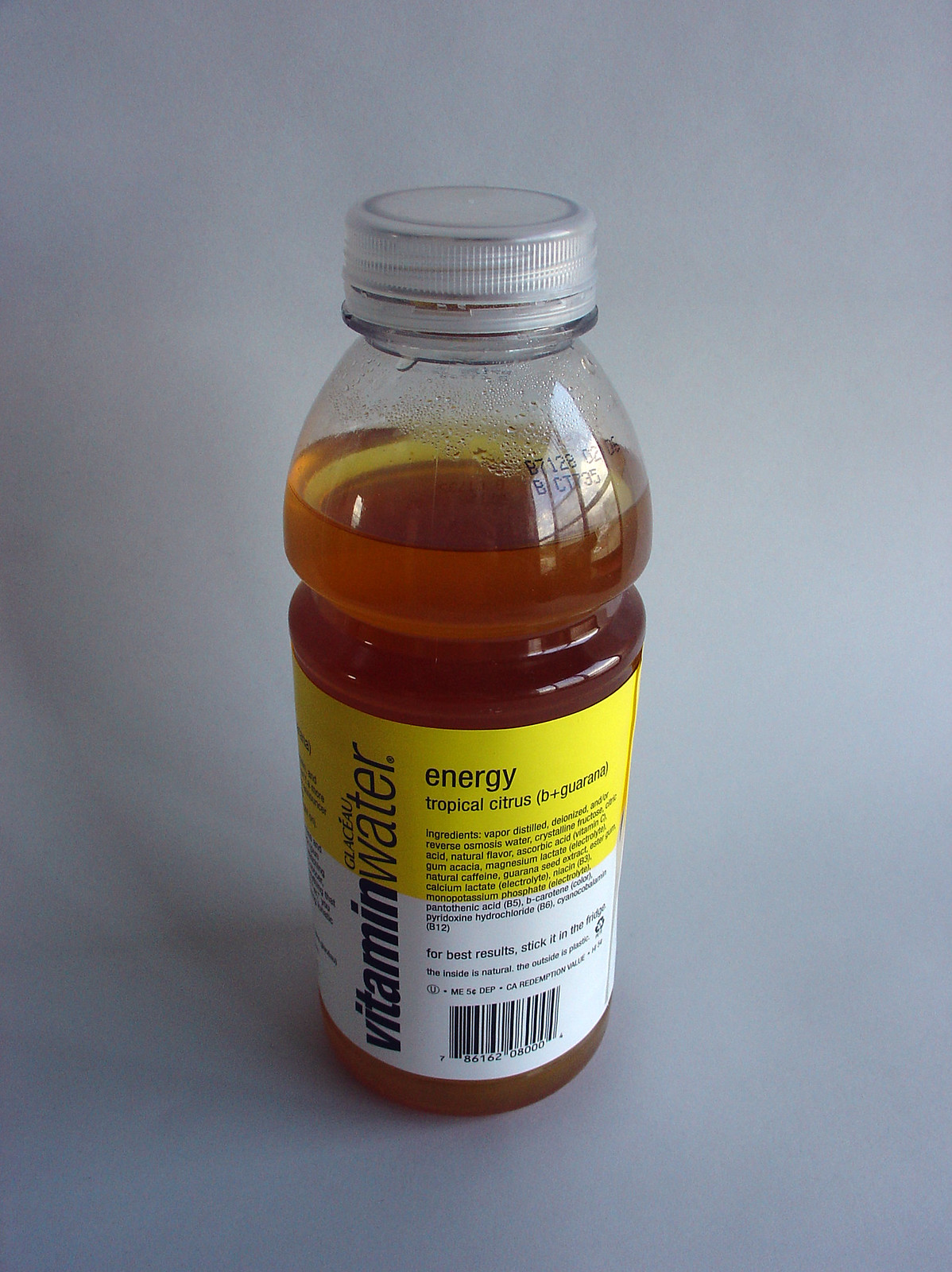This photograph showcases a bottle of Tropical Citrus Vitamin Water, partially consumed and positioned at an isometric angle against a pristine white background. The bottle, opened and with a few sips missing, displays a slight condensation on its interior, hinting at its refreshing coldness. The vitamin water, a warm tea-colored hue, complements the minimalistic setting, accentuating the product's vibrant and enticing appearance.